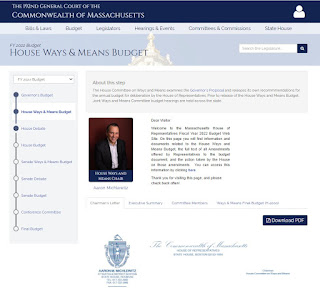A screenshot from the official Commonwealth of Massachusetts government website is displayed, specifically the House Ways and Means Budget section. The image features a quote from a speaker and a prominent "Download PDF" button for the budget report. On the left side of the screenshot, there's a navigation panel with a series of 10 dots, indicating different sections of the budget roadmap. The third dot is highlighted, signifying the current position in the navigation sequence. The quote from the speaker emphasizes the importance of adhering to the current budget and thanks readers for their diligence in staying informed.